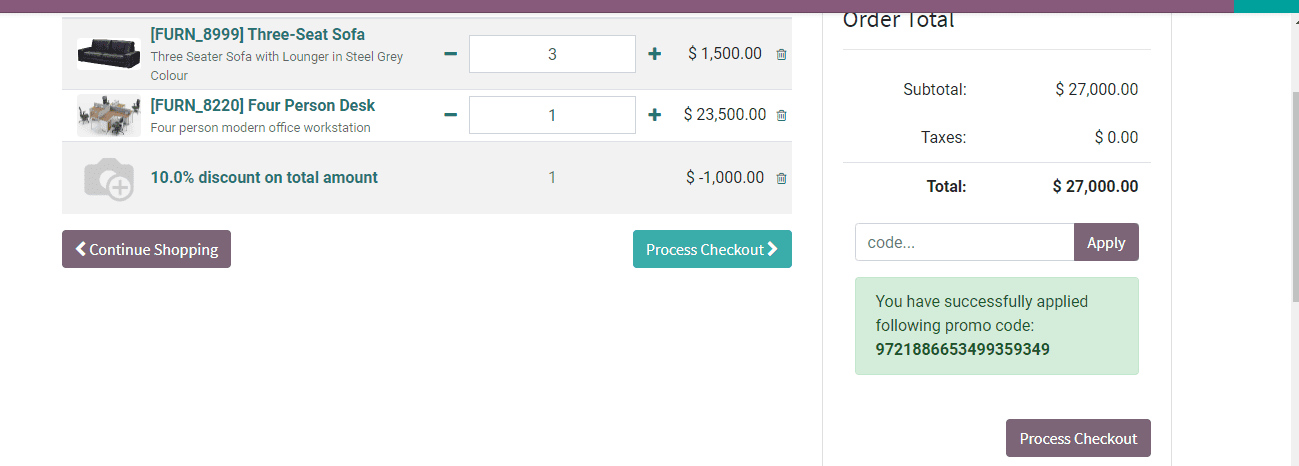This image is a detailed screen capture of a website's checkout page. At the top, a gradient bar transitions from burgundy on the left to a bluish-green color on the right. The page is divided into two sections: the main cart area on the left and the summary on the right.

On the left, there are three rows listing the products in the cart. Each product name is written in medium green text. The first row describes a "Pleasant Sofa" accompanied by an image of a black sofa on the left. Next to the sofa image, the quantity "3" is selected. The second row features a "Four-Person Desk," along with its corresponding image on the left. Below these listed products, there’s a grayed-out camera icon with a plus sign, indicating a 10% discount on the total. The price for the sofas is shown as $1,500, while the desk is priced at $23,500. A discount of $1,000 is applied to the order.

At the bottom left of the cart section, a blue button with white text prompts the user to "Process Checkout." Adjacent to it, a button with a marble-colored background and white text says "Continue Shopping."

On the right-hand side, a summary column is titled "Order Total." The subtotal is marked as $27,000, with zero tax, making the total also $27,000. Below this, a section allows for promo codes with an "Apply" button. At the bottom, there is confirmation that a promo code has been successfully applied, presented in a light green box. Another marble-colored button at the bottom right corner reiterates "Process Checkout."

The comprehensive layout and clear detailed elements ensure a user-friendly checkout experience.